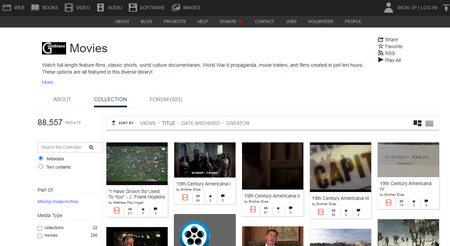The image depicts a web page titled "Google Movies" with the recognizable Google logo in the top left corner followed by the word "Movies." Below this title, there's a block of text that is too small to discern. Moving further down, the page features several tabs labeled "About," "Collection," and potentially "Forums," though the text is difficult to read due to its small size.

Under these tabs, a number is displayed prominently: "88,557." There is additional minor text following this number, but it remains unreadable. Beneath this section, there appears to be a filtering or selection menu, likely intended for navigating the movie collection; however, the options within this menu are indistinct.

Scrolling down, there is another bar with options labeled by categories such as "Date," "Approved," "Views," "Title," and "Creator," but, again, these labels are hard to read clearly. Finally, the main content of the page seems to be a display of movie thumbnails. Each thumbnail is accompanied by text that is largely indiscernible due to its small size. One thumbnail hints at the word "Capit," possibly "Capital," but is cut off. Another thumbnail is just text on a white background. Each thumbnail has icons below it, which seem to be thumbs up, thumbs down, and possibly a comment button, but the icons are not clear enough to be certain.